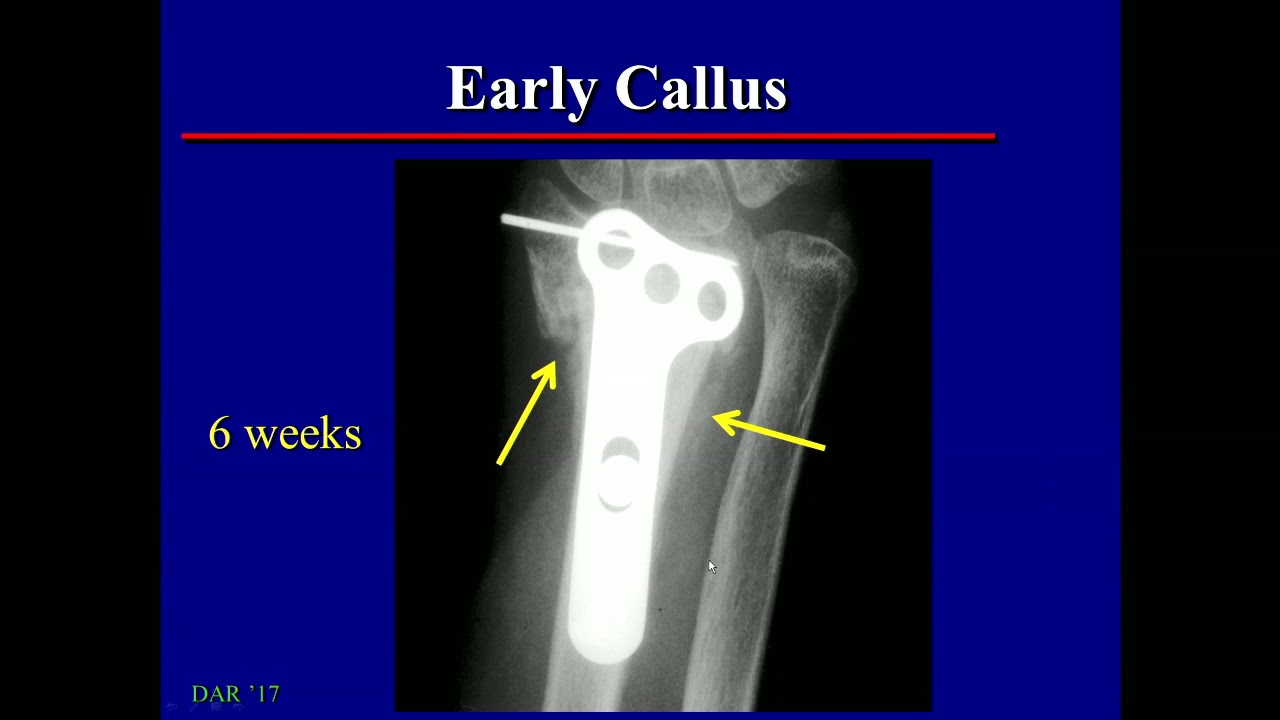The image features an x-ray with a predominantly blue background, bordered by black stripes on the left and right sides. Central to the image is an x-ray of leg bones, likely depicting the knee joint. The x-ray reveals two bones side by side, with one bone larger than the other. The knee joint appears rounded, indicative of either the early stages of healing or growth. Above the x-ray in white Times New Roman font is the text "early callus," underlined by a solid red line. Further down the image, "six weeks" is displayed in yellow text, also in Times New Roman, accompanied by two yellow arrows pointing towards a metal plate and screws affixed to the bone, illustrating the healing process. Additionally, the bottom-left corner of the image shows the text "DAR 17" in green, noticeably smaller than the other text. The metal plate within the bone is shaped somewhat like a key, with three circular holes at the top.